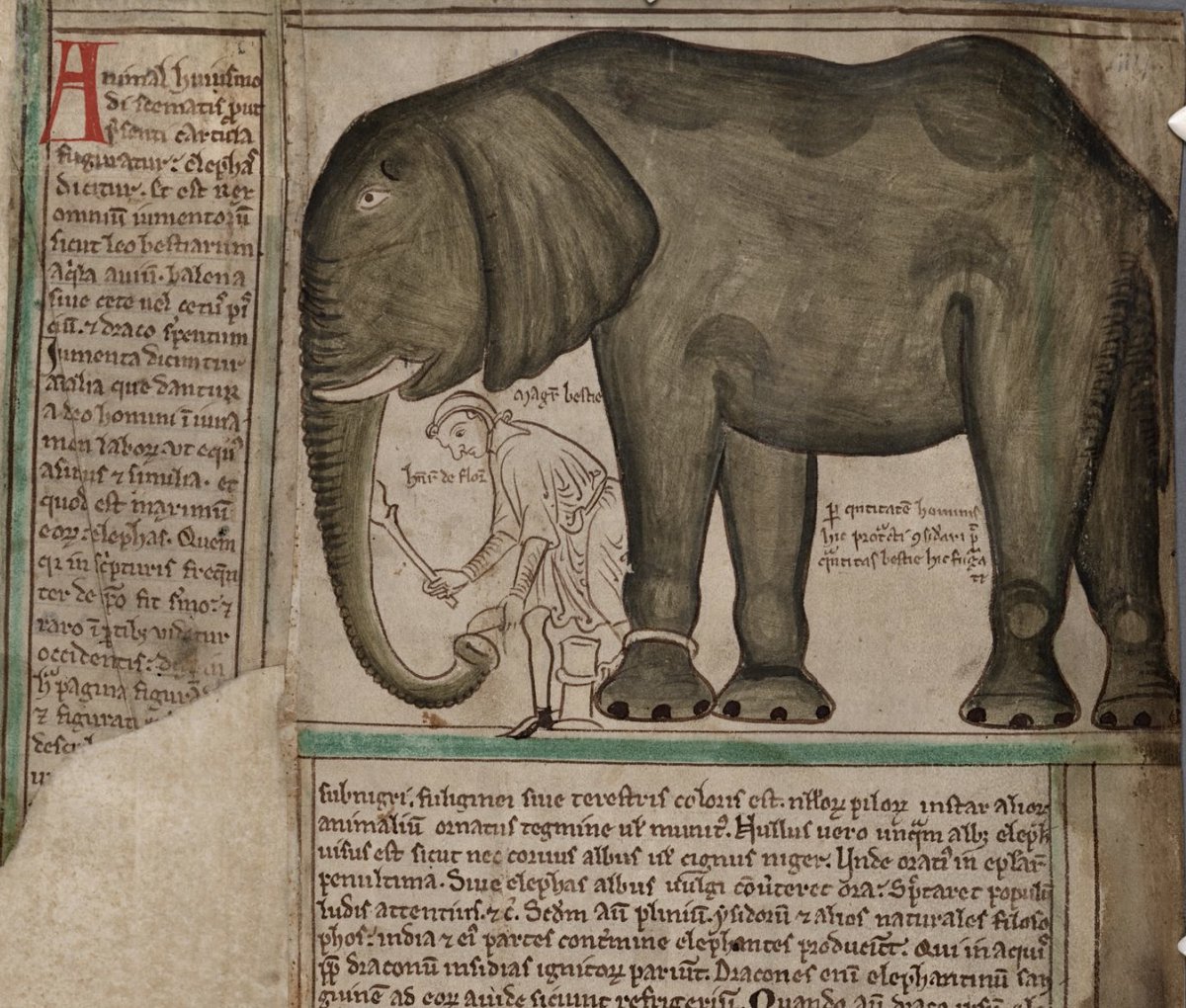This image features a detailed folio from a medieval manuscript, rich in Latin text and elaborate illustrations. Dominating the center of the page is a painted drawing of a large gray elephant, magnificently detailed with visible striping on its trunk and ears. The elephant is looking toward the Latin script positioned to its left. Below its head, a man wearing a hat appears to be engaged with the elephant's trunk, possibly applying or cleaning something with various tools. His black shoes and a single visible leg add to the scene's intricacy. The elephant's front left ankle is shackled to a pole extending from the ground, and more Latin text is nestled between its legs. Notable is the small hole in the bottom left corner of the manuscript, testifying to its ancient and well-worn nature. The manuscript page itself is a dingy beige-gray, with a striking red initial letter and some blue watercolor strippings adding a touch of color amidst the otherwise aged and damaged background.